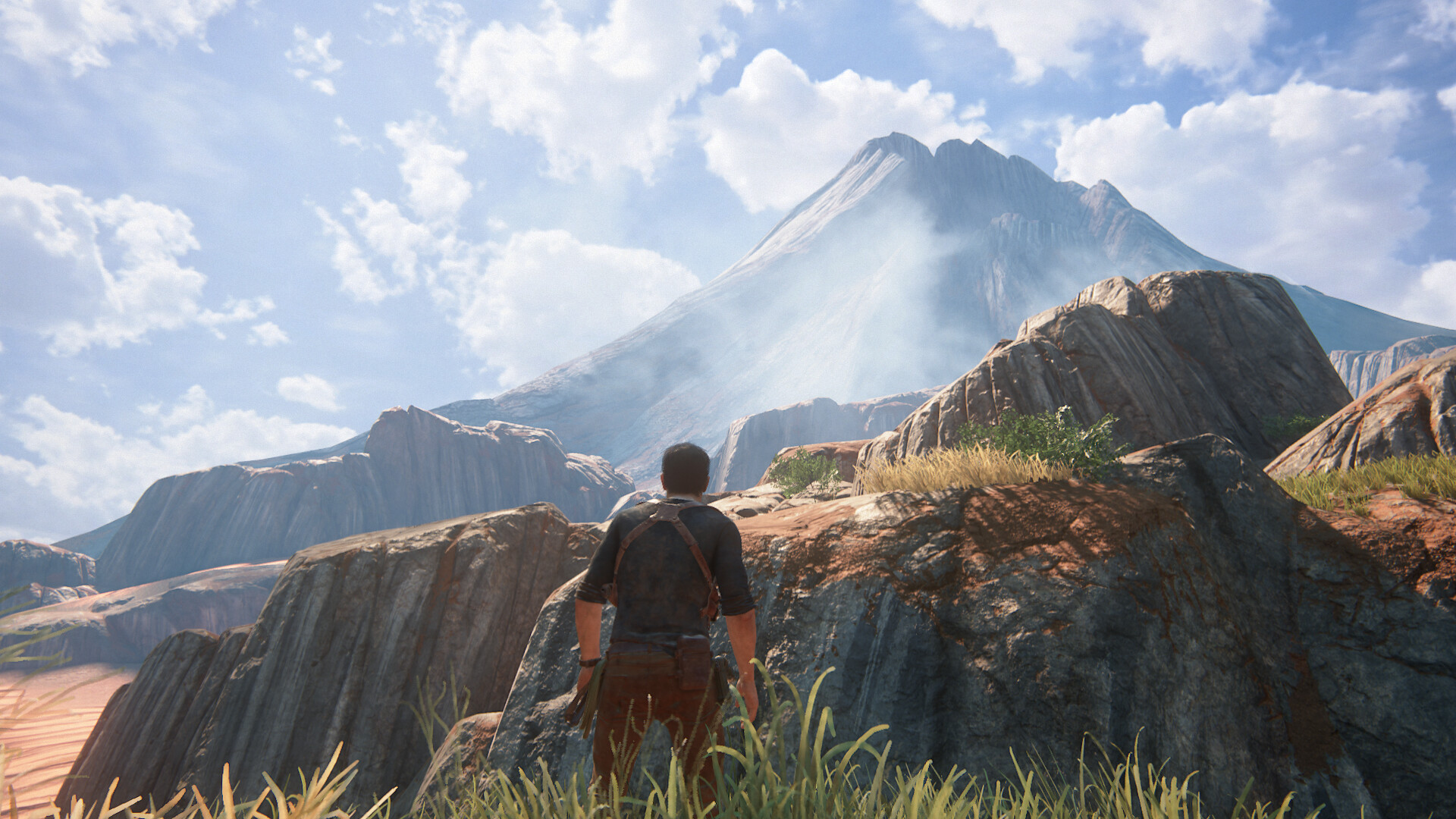A scene from a video game depicts a character standing outdoors amidst a rugged landscape. The foreground features a grassy terrain interspersed with weeds sprouting from the bottom of the frame. Central to the composition is a male figure, viewed from behind, dressed in brown pants and a long-sleeved shirt with rolled-up sleeves. His outfit includes a leather harness strapped across his back, and he sports dark hair. Directly ahead of him looms a prominent gray rock formation, tinged with brown at the top and speckled with dry grass and weeds.

Flanking this primary rock are two additional large rock formations, one on either side. Beyond these, a smaller rock outcrop is visible in the middle ground. Dominating the background is a towering mountain, rising majestically towards a light blue sky adorned with fluffy white clouds. The interplay of natural elements creates a layered and immersive environment, capturing the rugged beauty of the game’s setting.